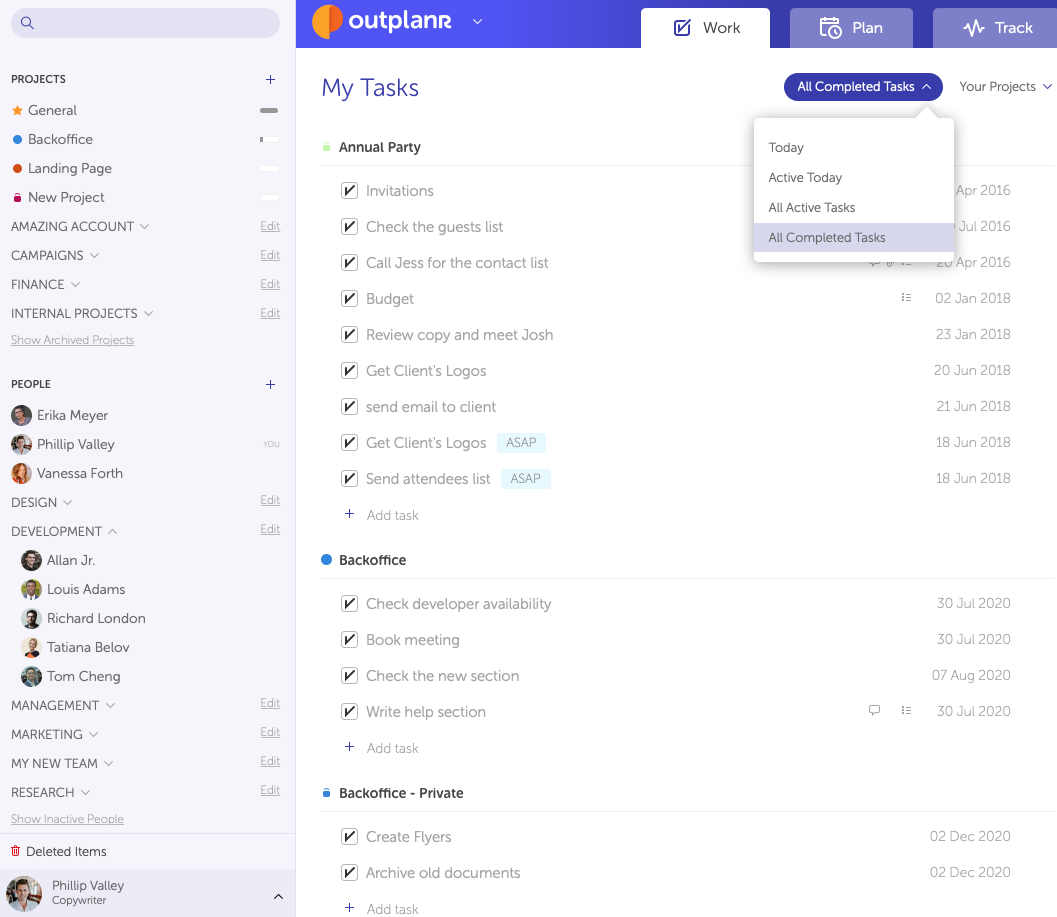This screenshot captures a workspace within a software application named Outplan R, primarily used for project and task management. The interface features a light grey vertical sidebar on the left, labeled "Projects" at the top. Beneath this label, various project categories are listed in the following order: General, Back Office, Landing Page, New Project, Amazon Account, Campaigns, Finance, and Internal Projects.

Additionally, the screenshot displays user profiles that are visible to Erica Mayer, Philip Vallee, and Vanessa Forth, organized under development sub-sections including Alan Junior, Louis Adams, Richard London, Tatiana Belov, and Tong Cheng. There are also category sections for Management, Marketing, My New Team, and Research. At the very bottom of the sidebar, there is a small profile picture of Philip Vallee, identified as a copywriter.

The application’s branding, Outplan R, is positioned at the top with a logo consisting of a light orange half-circle paired with a smaller dark orange half-circle, accompanied by the name "Outplan R" where the "R" is capitalized. Additionally, there is a small white cap icon on a blue background.

The main content area of the interface is currently displaying the "Work" tab, part of a trio that includes "Plan" and "Track" tabs. In the "Work" tab, a list titled "My Tasks" enumerates specific tasks alongside their respective dates. Tasks include:
- Invitations
- Check the Guest List
- Call Jess for the Contact List
- Budget Review
- Copy and Meet Josh
- Get Client's Logo
- Send Email to Client
- Get Client's Logo (appears twice)
- Send Attendees List ASAP

Furthermore, under the "Back Office" section, there is a private task list that includes:
- Create Flyers
- Archive All Documents

These tasks are presumably to be completed or marked as done by the user.